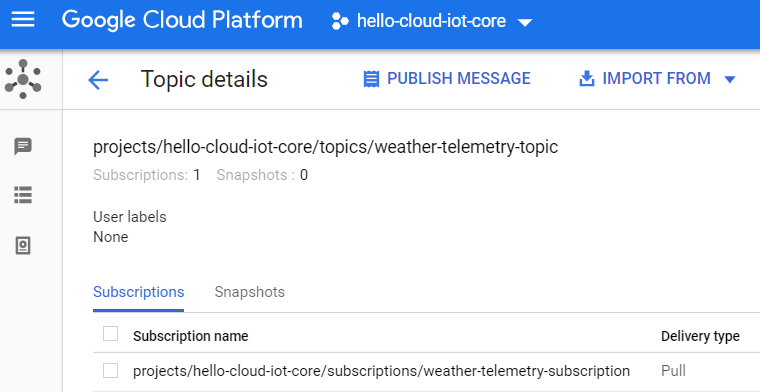The image depicts a user interface belonging to the Google Cloud Platform, specifically showcasing the "Hello Cloud IoT Core" dashboard. On the left-hand side, there is a hamburger icon used for navigation. The center of the image features a distinctive graphical element: a main circle connected by lines to three surrounding circles, with additional smaller circles interspersed between them.

On the upper right corner, there is a chat icon, followed by three squares each containing three rectangles, positioned vertically. To the far right are various icons, including one that resembles a certificate, depicted as a rectangle with a small square and a line within it.

At the top of the interface, there are tabs labeled "Topic Details," "Publish Message," and "Import From." The breadcrumb navigation reads: "projects/hello/project/hello-cloud-IoT-core/topics/weather-telemetries-topic." 

Additional details include:
- "Subscriptions: 1"
- "Snapshots: 0"
- "User Labels: None"
- "Subscriptions and Snapshots" 

This detailed interface appears to be part of the IoT (Internet of Things) management tools within Google Cloud Platform, providing detailed telemetry data and options for managing IoT device communication.